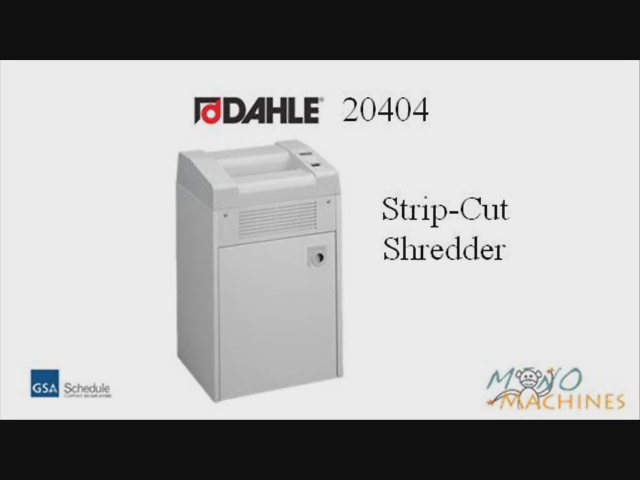The advertisement showcases the DAHLE 20404 strip-cut shredder against a white backdrop with black horizontal bars at the top and bottom. The brand name "DAHLE" is prominently displayed in black bold text, accompanied by its distinctive logo featuring a half-square in black and a round, red letter "D." The model number "20404" is positioned to the right in thin black text. At the bottom left of the image is a blue square with the white letters "GSA," and beside it, the word "SCHEDULE" appears in gray text with smaller, unreadable text beneath it. In the bottom right corner, there is the text "MANO MACHINES," with "MANO" in green and "MACHINES" in yellow, accompanied by an illustration of a monkey face for the letter 'O.' The shredder itself, depicted in the center, is gray and features long horizontal vents on the front and a panel that appears to have a lock mechanism, indicating it is a top-loading paper shredder.